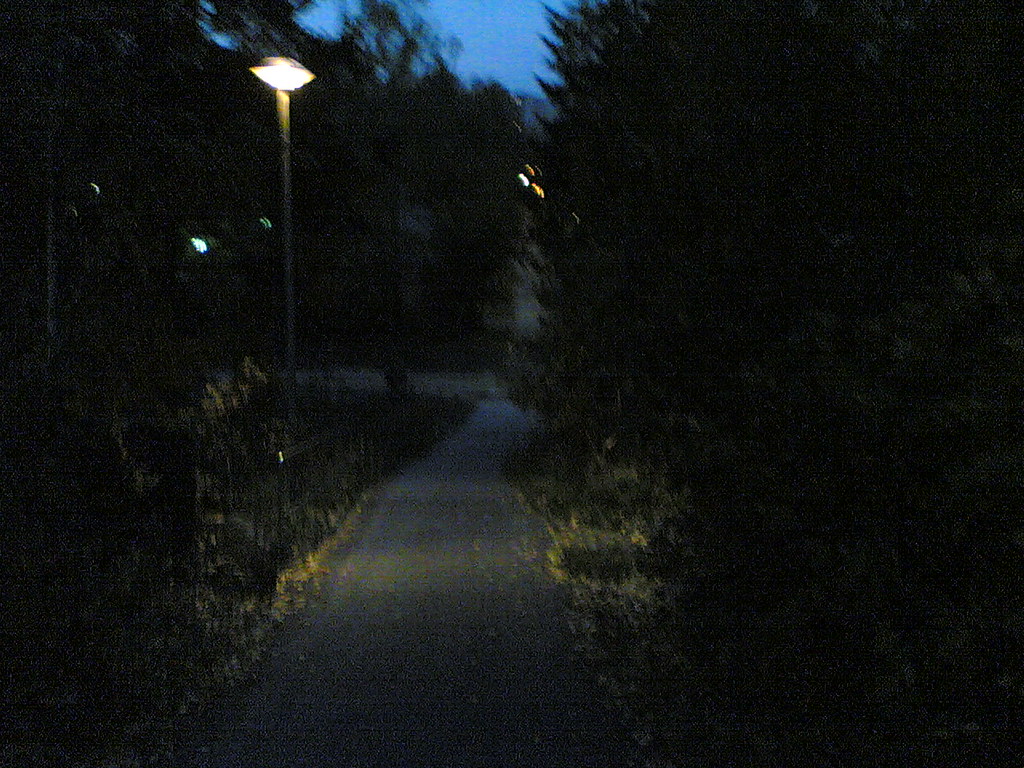This image captures a dimly lit, small asphalt footpath during late evening or nighttime. The sky in the distance shows a faint blue hue, indicating that the sun has already set. The path, which begins at the bottom center and leads to the middle of the image, is flanked by patches of grass and a variety of greenery. On the left side, a low black fence is visible, with shrubbery and bushes growing alongside it. A streetlight, resembling a UFO or oval shape, stands on a black pole along this side, casting a warm yellow light onto the path. The right side of the image is dominated by tall, bush-like trees and dense shrubbery that appear dark green to black in the low light. In the distance, the path seems to intersect with another path or a small road, partially illuminated by the lone streetlight. The overall scene is serene yet slightly eerie due to the sparse, dim lighting and the dense, surrounding foliage.